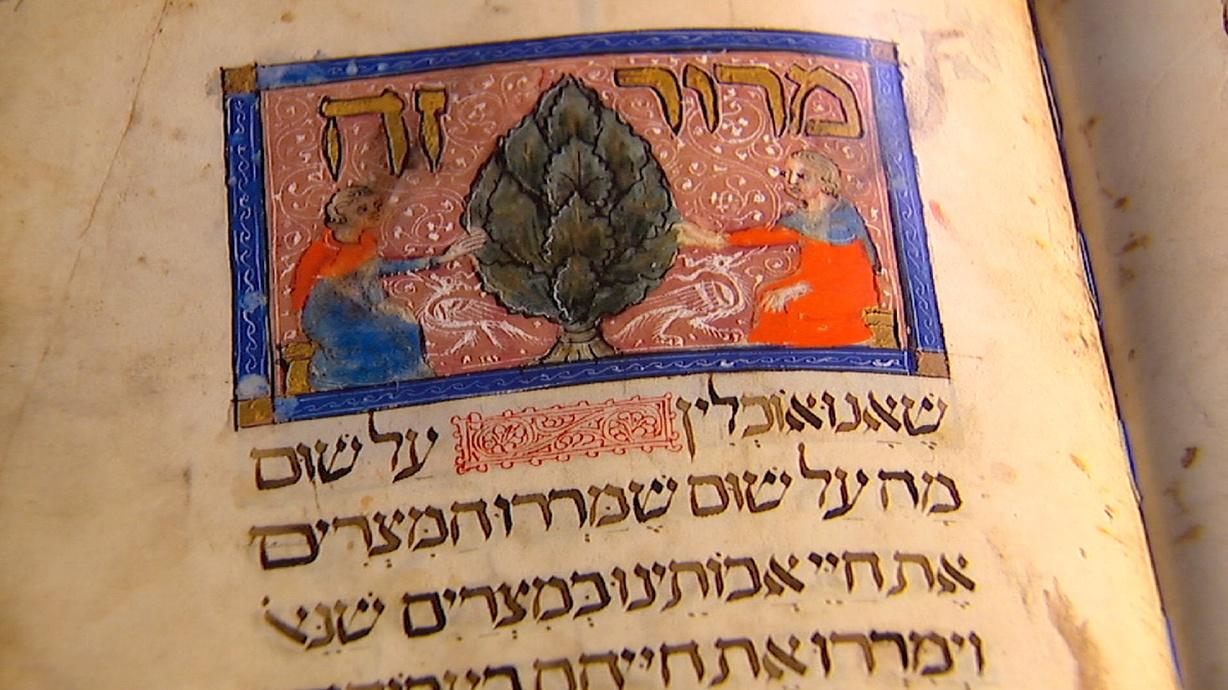This image features a rectangular artwork bordered in rich hues of dark purple or blue, each corner adorned with a brown square. The central illustration rests upon a textured brownish-red background decorated with white wavy lines. Dominating the composition is a tree-like figure, reminiscent of an artichoke, rendered in varying shades of dark gray. Flanking this central figure are two human forms, each reaching towards the tree. The figure on the right is dressed in a red garment with a blue collar, extending their right hand; the figure on the left wears a blue garment with a red collar, stretching their left hand towards the tree. Above the illustration lies an area of Hebrew script, while below the image are four lines of additional Hebrew text in brown, with a notable red feature prominently placed in the middle of the top line. The surface surrounding the artwork is a light brown or tan, lending a rustic feel to the overall presentation.